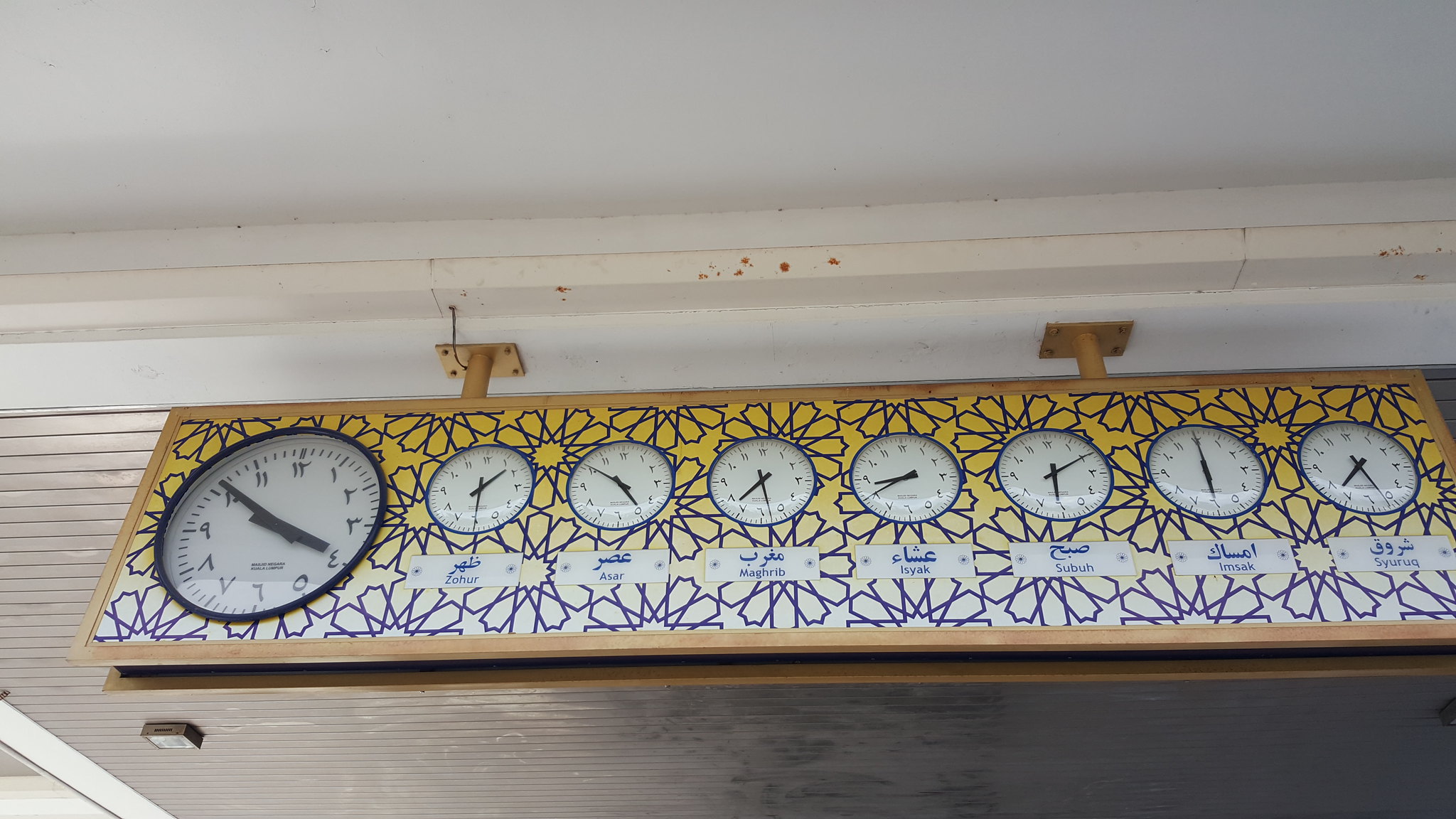The image showcases a meticulously detailed installation of clocks, featuring a long, rectangular frame securely fastened to the ceiling. The frame, crafted from a golden-brown metal, boasts intricate geometric circular patterns in black against a yellow backdrop. Within the frame, eight round clock faces are prominently displayed. To the left, a larger clock with bold black hands stands out, while the remaining seven smaller clocks are evenly spaced, each indicating the time for a different global location. This arrangement offers a striking visual representation of time across various cities, underscored by the elegant and coordinated aesthetic of the design elements.